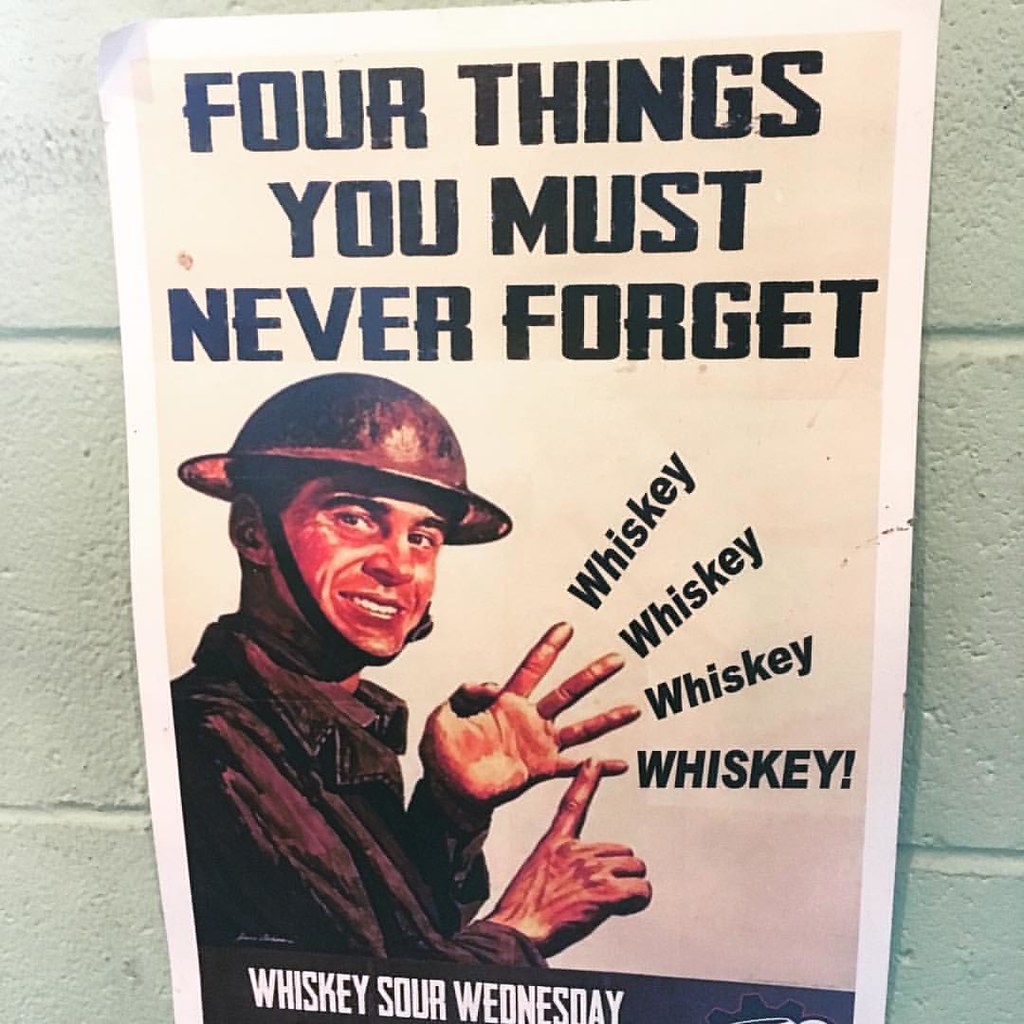The image captures a photo of a poster taped to a brick wall painted off-white, suggesting the setting is an institutional building like a school. The poster features a white border and a tan background. Dominating the poster is a detailed, smiling illustration of a military officer wearing a traditional army helmet with a chin strap. His sunburned face and dark eyes are prominent features. The officer, clad in a dark uniform, holds up his left hand, displaying four fingers. His other hand points to his pinky, emphasizing each of his fingers with the word "WHISKEY" in bold black text, and the final "WHISKEY" accompanied by an exclamation mark. Above this illustration, the text reads in large black type: "Four things you must never forget." A black banner at the bottom of the poster proclaims "WHISKEY SOUR WEDNESDAY" in white text, indicating the poster promotes a whiskey-related event. The poster appears to be about 12 to 14 inches tall.